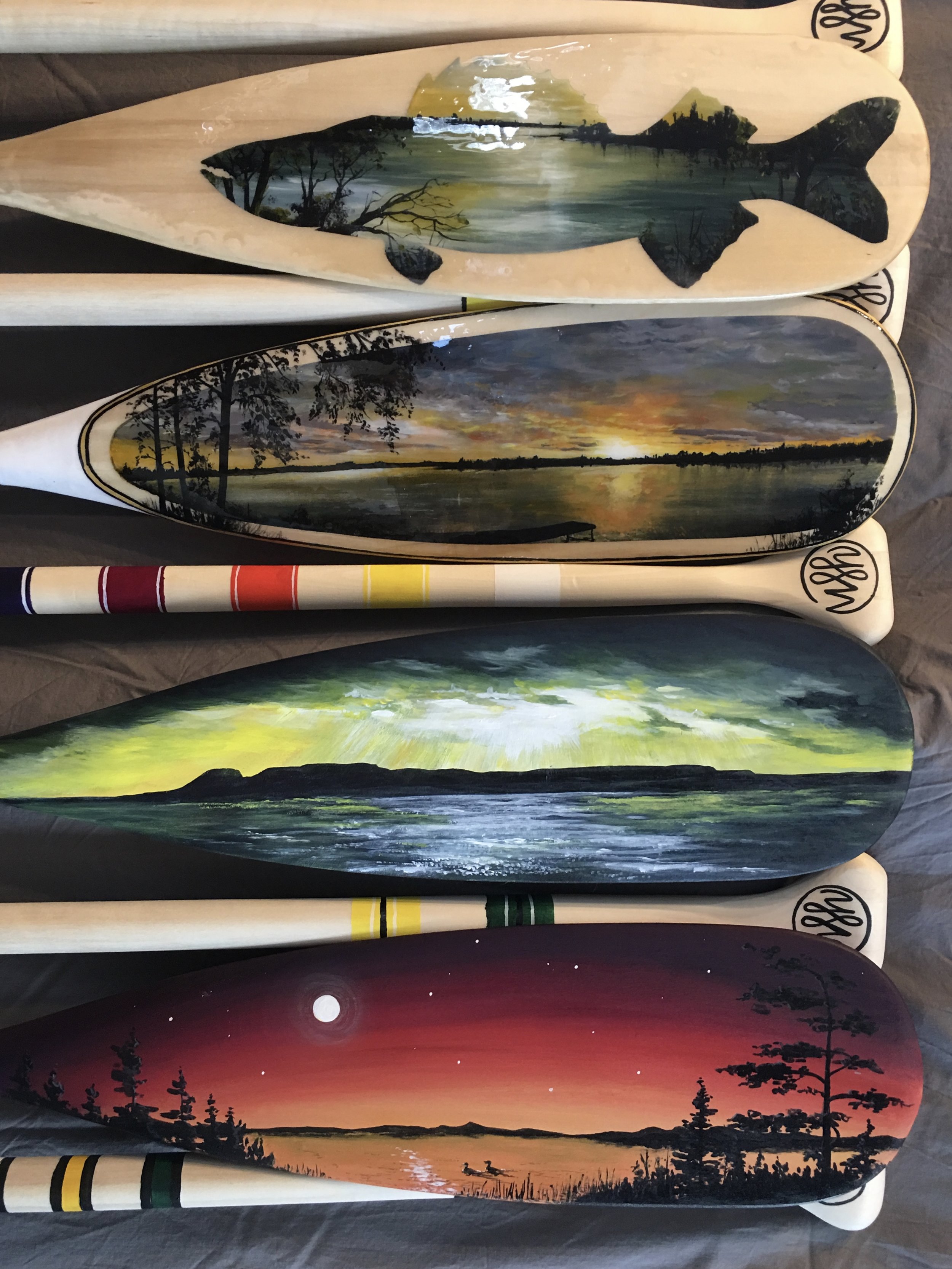In this image, a collection of light beige-colored wooden paddles are artistically laid out against a grayish-green background. Some of the paddles feature intricate hand-painted scenes. At the top, there's a paddle with a detailed painting of a green trout facing left, surrounded by tree branches and a lake. Below it, another paddle showcases a serene lakeside sunset with trees framing the scene on the left. The third paddle depicts a vibrant blue ocean bordered by mountains under a greenish sky. The next features a stylized desert-like landscape under a striking red sky, dotted with scattered white stars and a large white moon on the left. This paddle also has trees on either side, adding a touch of nature to the arid scene. All paddles have a natural wood finish with a stain that enhances their beauty, particularly the lowest one, which stands out for its vivid, detailed depiction of the night sky with stars and the moon.